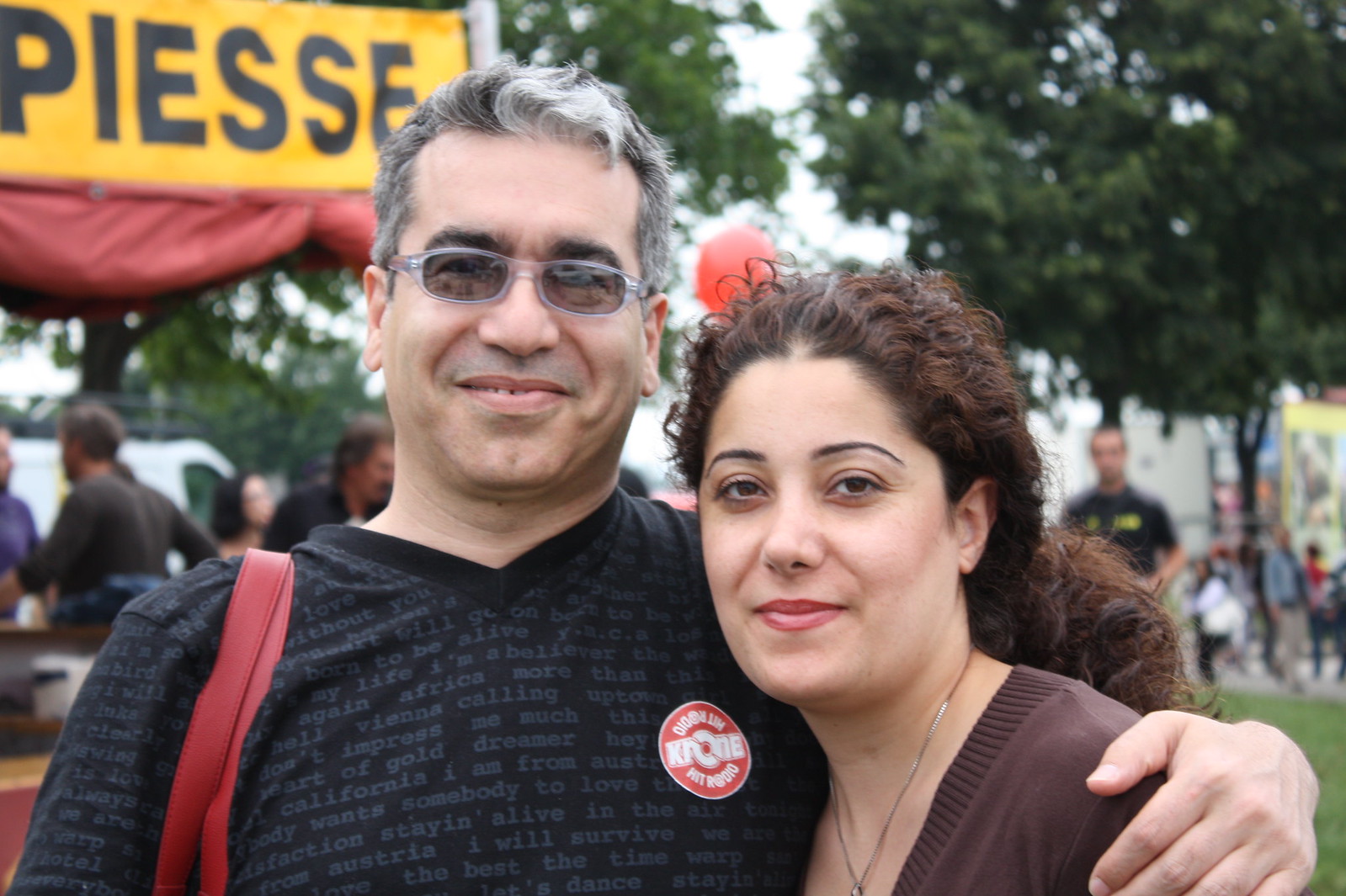In the image, a man and a woman are posing outdoors, seemingly at a fair or similar event. The man, who appears to be Latino, is on the left. He has short, graying black hair and wears tinted sunglasses. His outfit consists of a black v-neck shirt adorned with a red and white circle on the left chest, and he has a red strap slung over his right shoulder. He's smiling and has his arm around the woman beside him. She has long, dark curly hair and is wearing a brown sweater with a plunging neckline, complemented by a necklace. To the right, she is slightly smiling. Behind them, people can be seen sitting at tables and walking around on the grassy area. There are trees in the background and a yellow sign with black writing and a red valance hanging below it. The scene is set under a cloudy sky, adding to the bustling yet relaxed outdoor atmosphere.